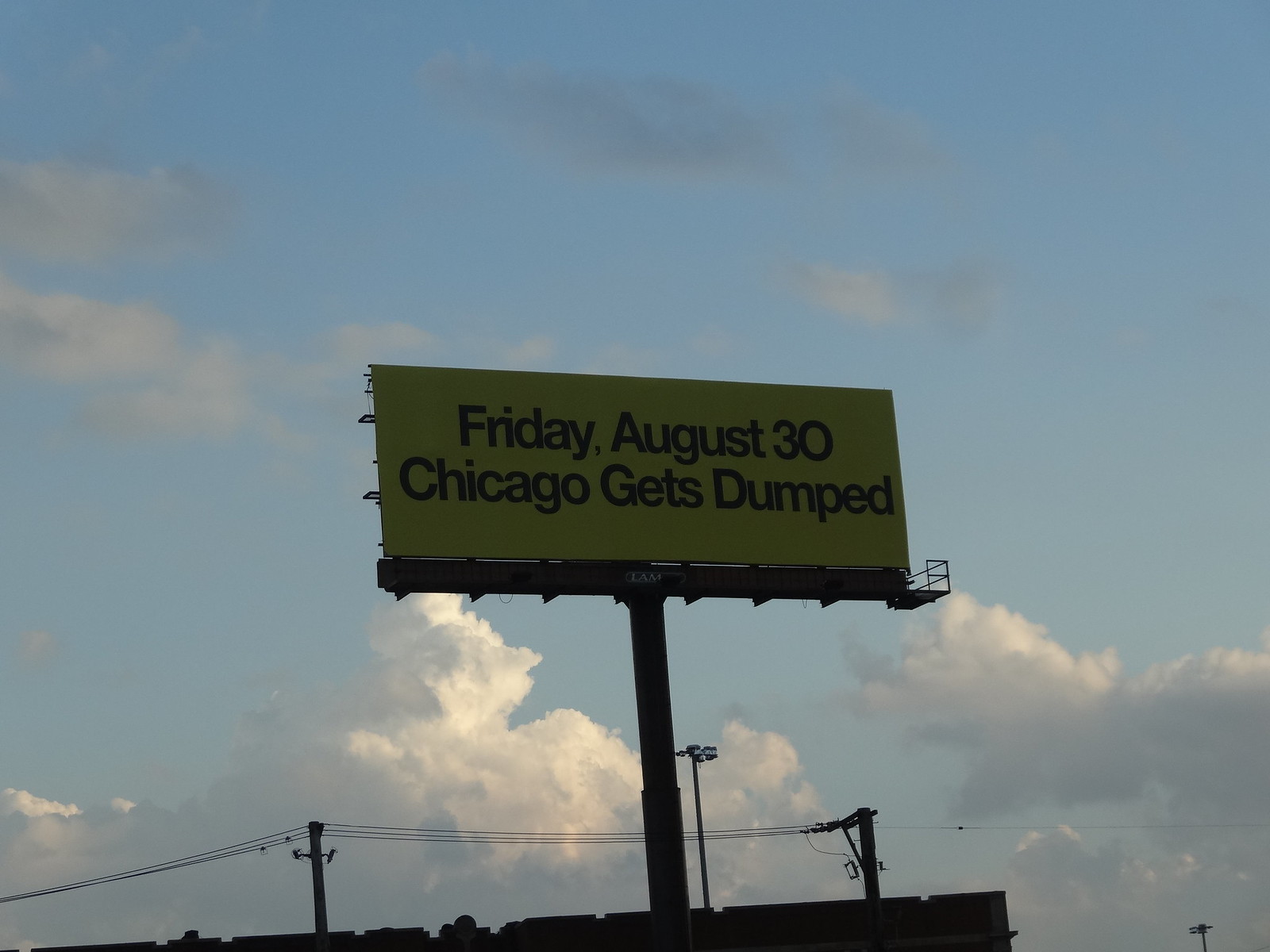A photo taken outdoors during a cloudy day reveals a sky densely packed with clouds. The image centers on a prominent yellow billboard with dark writing that reads, "Friday, August 30, Chicago Gets Dumped." At the bottom edge of the photo, the top of a building is faintly visible, grounding the urban scene. The focus remains firmly on the striking billboard against the overcast backdrop.